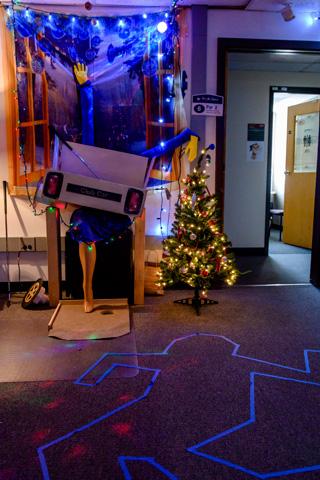The photograph depicts a dimly lit room with multiple points of interest. The floor, which appears to be either tile or carpeted, features a large chalk or blue tape outline of a person, reminiscent of a crime scene. Along the wall, there is a small, illuminated Christmas tree adorned with white lights and ornaments. To the left of the tree, there is a piece of exercise equipment or a decorative element resembling the back of a truck with two headlights. Standing behind this metallic structure is a figure of a woman in a blue dress with one leg raised, one arm pointing upwards, and the other arm extending to the right. This figure, set against a bright blue backdrop with lights, appears to be a decoration or possibly an art installation. On the right side of the room, an open wooden door reveals a view into another space, which may be an office, indicated by the presence of a chair and additional lighting from the adjacent room.